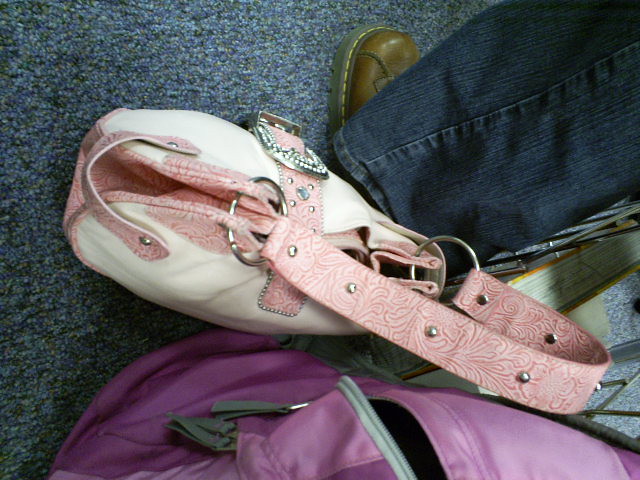This detailed top-down photograph captures a visually intriguing scene set against a blue and mottled black rug. At the center lies a striking white purse adorned with elaborate pink detailing, including a wide pink shoulder strap with silver studs and a strap down the front secured with a silver buckle. To the lower right, a partially visible purple backpack with an open zipper adds a splash of vibrant color. In the top left corner of the image, a person's leg clad in blue jeans and a brown boot, possibly a Doc Martens, makes an appearance, suggesting their presence in the scene. The photograph, rendered in realistic color and landscape orientation, showcases the intricate textures and hues of the objects within the frame.